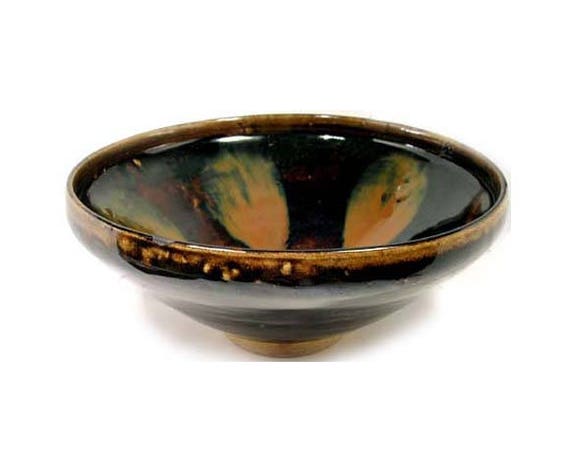This detailed close-up image depicts a handcrafted ceramic bowl with a rich, dark brown glaze accented by lighter brown hues. The bowl, positioned on a completely white background, features a distinctive thin, yellowish-brown foot that supports it. Its rounded form is not entirely smooth, with the lip displaying slight imperfections that add to its charm. The interior of the bowl is equally fascinating, with a glazed brown surface adorned with leaf-shaped imprints in tan, rust, and greenish tones, hinting at meticulous decoration. The inside also presents hints of darker colors and gold accents between the imprints, suggesting a thoughtful, artisan touch. Likely hand-fired, the bowl, casting a light shadow on its white surface, seems to be intended for decorative purposes rather than practical use.